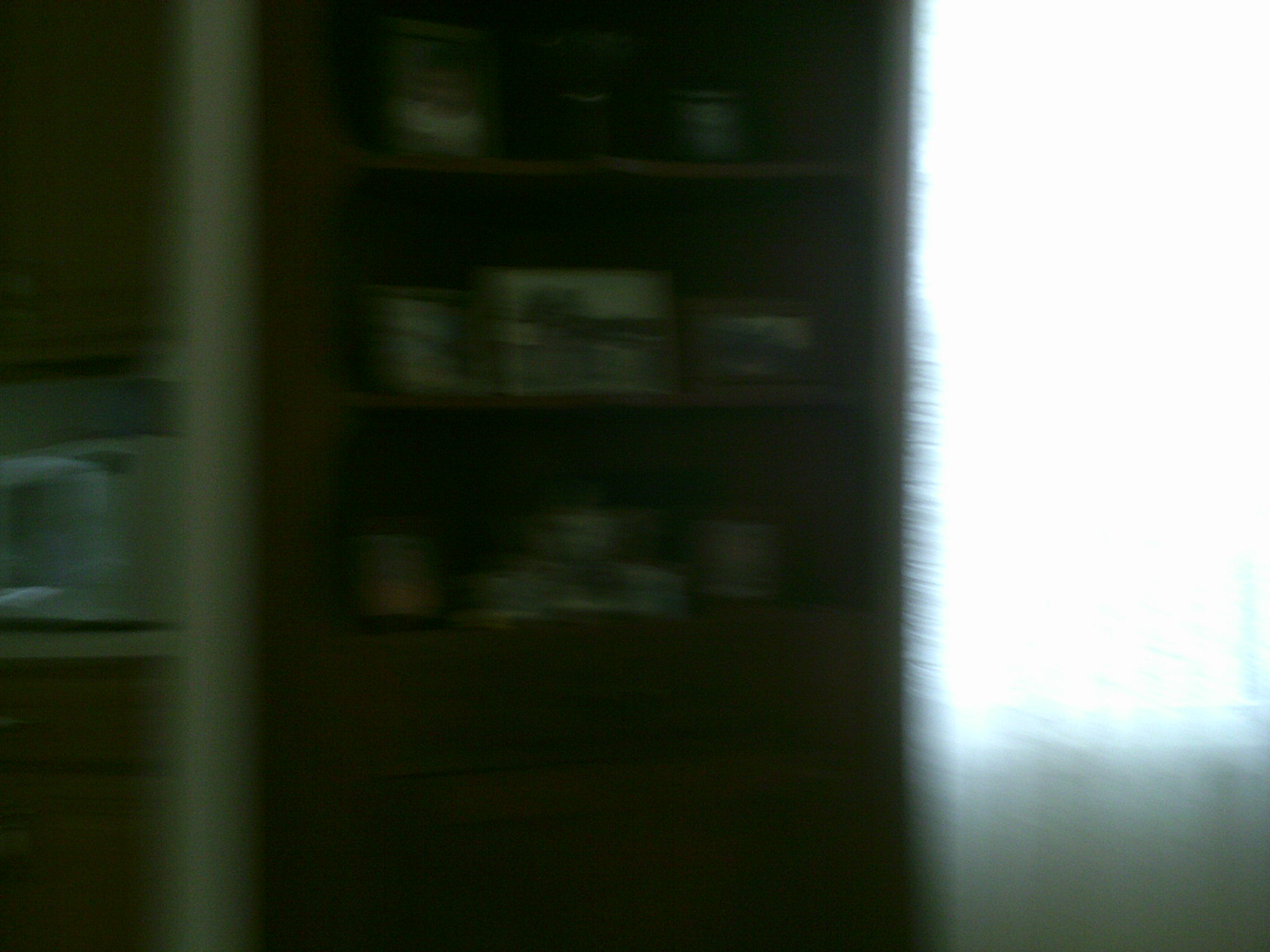The image, though blurry, captures a brown cabinet situated towards the left center. The cabinet features three open shelves above a closed door at the bottom. Each shelf holds various items: the middle shelf hosts three picture frames, one in the center, one on the right, and a cup on the left of the central frame. The top shelf displays another picture frame on the left, a potted plant in the center, and a cup on the right. The bottom shelf contains white cups and bowls dispersed across it. On the far right side of the image, a bright white light filters in through a window.